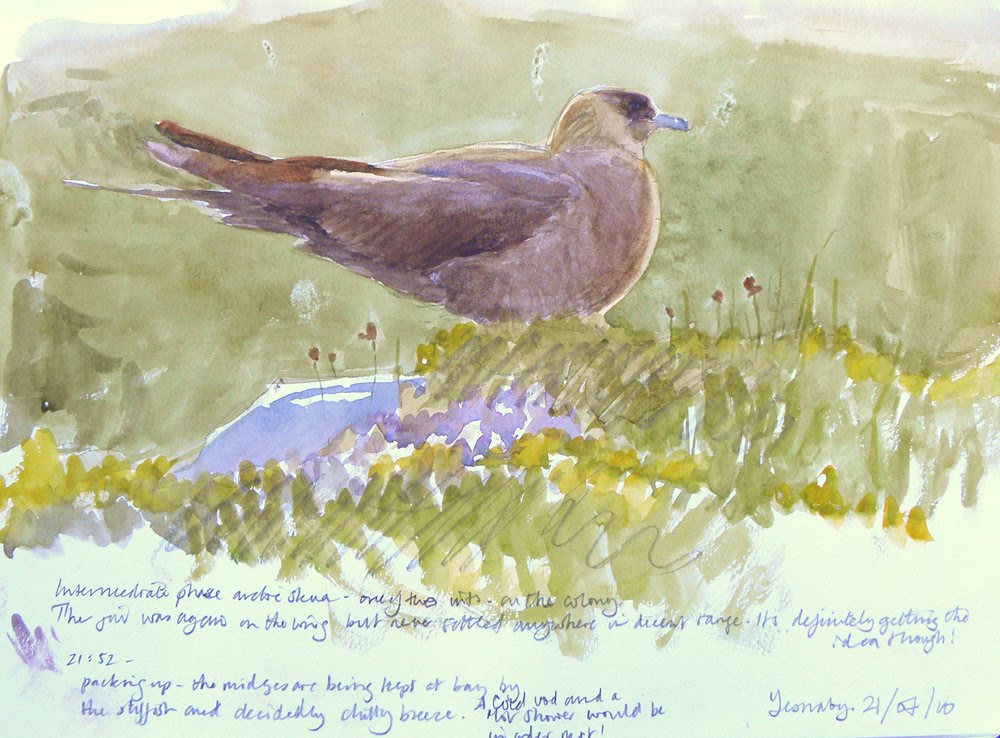The painting depicts a brown bird facing the right side, standing on green grass beside a puddle with a blue hue that matches the bird's blue beak. The bird's feathers are dark brown, and the surroundings include a few flowers both in front and behind it. The background is predominantly green. Below the image, there is a significant amount of handwriting in script, which is illegible, except for the date "21/07/10" in the lower right corner. The script seems to be someone's handwriting, possibly a signature, adding a personal touch to the artwork.